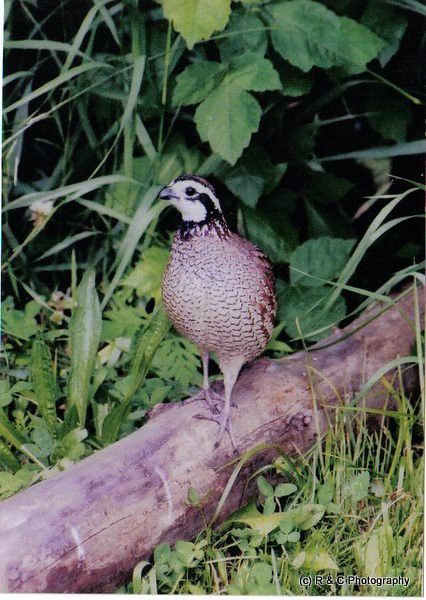This close-up photograph captures a lovely small bird perched on a fallen tree branch amidst a lush, green landscape. The bird, which is primarily a darker brownish color with accents of white, has a distinctive white face with black trim and a black beak. Its head, positioned to showcase a direct view of its left eye, is relatively small compared to its body and adorned with black streaks under the eye. The bird's feet, with claws spread out, grasp the branch, which seems to have a purplish hue and is settled into a grassy area. The background and foreground are filled with greenery, shrubbery, leaves, and twigs, suggesting an outdoor setting possibly resembling a greenhouse or a shaded locale. In the bottom right corner of the image, the text "Copyright RNC Photography" is clearly visible in black, signifying the ownership of the photograph.